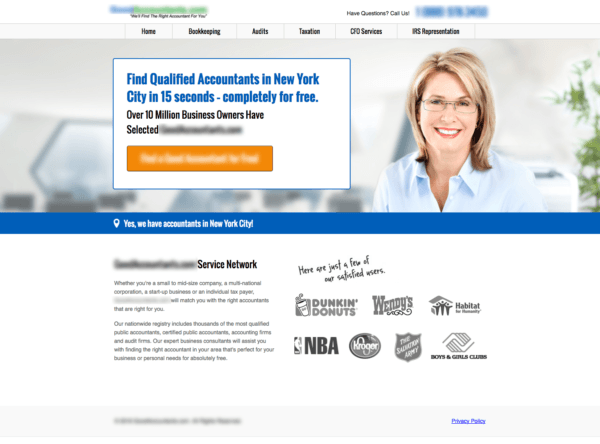The webpage appears to belong to an accounting services provider, with certain business details intentionally blurred out. The top of the page features a standard navigation bar with sections labeled: Home, Bookkeeping, Audits, Taxation, CFO Services, and IRS Representation. Spanning the width of the screen is an image depicting a professional setting. On the right side of the image is a smiling woman with blonde hair and glasses, dressed in a white shirt. Behind her, some foliage is visible, but the rest of the background is blurred.

Overlaying the image on the left is a text box containing the headline, "Find qualified accountants in New York City in 15 seconds, completely for free." The text continues, stating that "Over 10 million business owners have selected" followed by blurred content and an orange button that is also blurred out.

Below the banner image, a blue bar reads, "Yes, we have accountants in New York City." Under this, there's a mention of a service network, blurred out, accompanied by an unreadable paragraph of text. To the right, there is a section showcasing logos of reputable customers, such as Dunkin' Donuts, NBA, Kroger, Wendy's, Salvation Army, Habitat for Humanity, and Boys and Girls Clubs.

At the bottom of the page, there is grayed out text along with a link to the company's privacy policy.